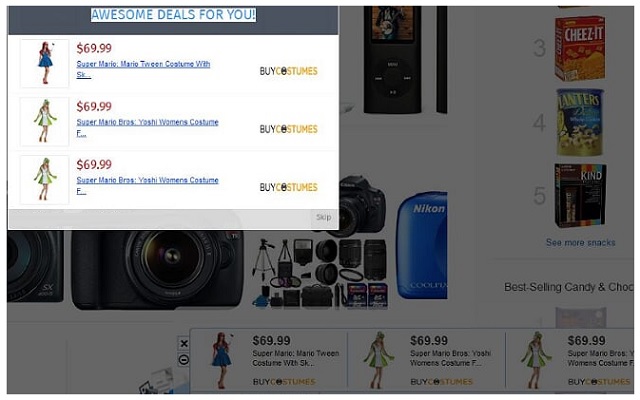The image is a screenshot from an e-commerce shopping website that features a diverse range of products, including food, electronics, and clothing. The focal point of the image is a pop-up window located in the upper left quadrant, displaying three dresses themed after Super Mario Bros., each priced at $69.99. The dresses come in three designs: one in blue and two in green. The pop-up also mentions "BuyCostumes.com," suggesting that the website might be acting as an intermediary, directing users to other outlets for their purchases.

The rest of the image, although darker due to the focus on the pop-up, reveals a glimpse of various product categories. On the right-hand side, there is a column dedicated to best-selling snacks, candies, and chocolates, with items ranked as 3, 4, and 5. Item 3 is a red Cheez-It box, item 4 is a blue Planters box, and the details for item 5 remain unreadable. To the left of this column, a range of electronics can be seen, including cameras and MP3 players, indicating that the image might be from an older period.